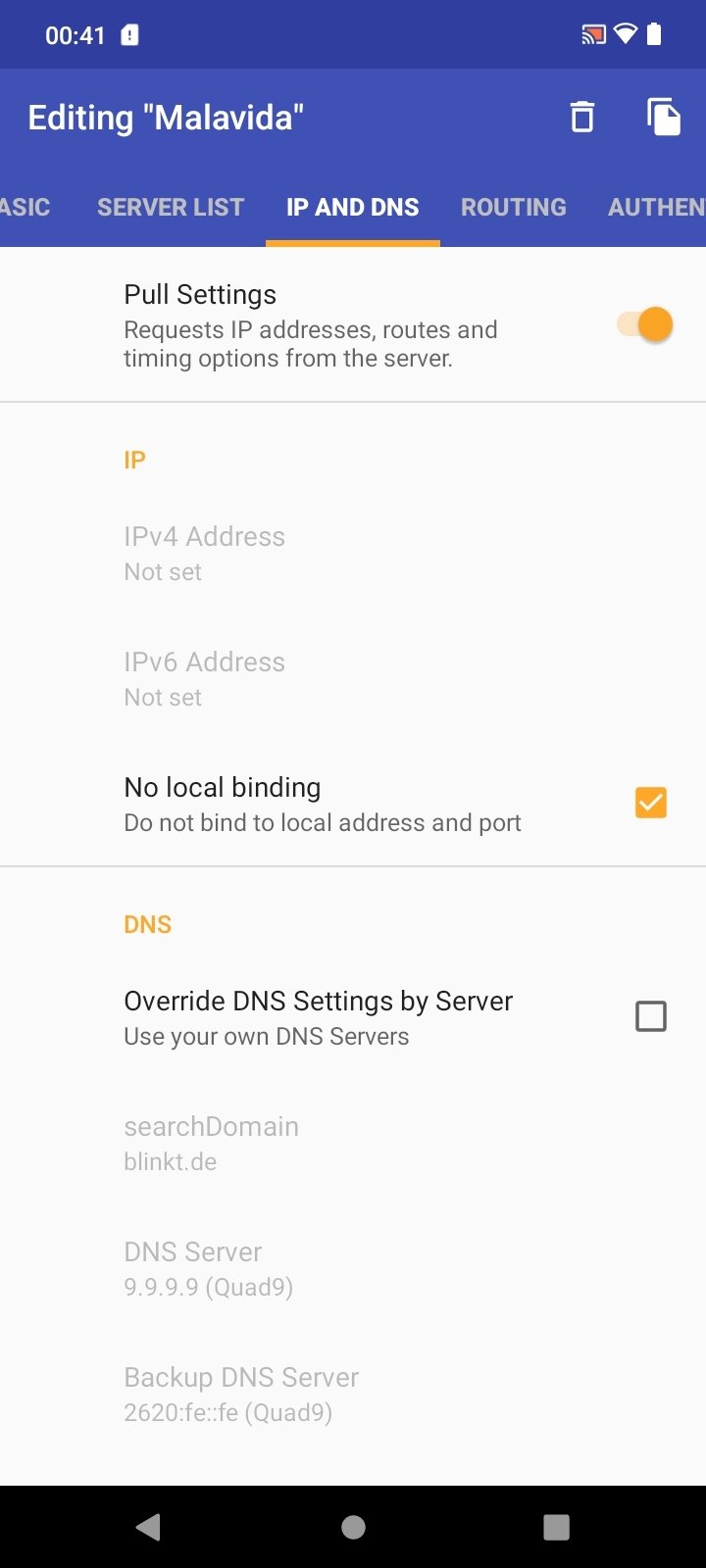This image is a vertically oriented rectangular screenshot taken from a cell phone. In the upper left-hand corner, the screen displays the time "19:26" in a white font, set against a dark blue horizontal background. Directly beneath this, another blue horizontal section reads, also in white font, "editing quotes". Following this, there's a string in lowercase letters enclosed in quotes: "vpniify".

Below this section, a menu with several options is visible. The first menu item is partially cut off on the left and is grayed out, showing only the ending letters "TION", followed by "/ encryption". The second option, which is selected, is "ADVANCED" in all capital letters, highlighted by a mustard yellow underline. Next to it is another option, "ALLOWED APPS", also in all caps.

Beneath these menu options, there's a heading in yellow text that reads "Behavior". Below this, in bold, the word "persistent" is written, followed by "tun" in lowercase letters. In a smaller, lighter font, the description reads: "Do not fall back to no VPN connection when OpenVPN is reconnecting." To the right of this description is an unchecked square checkbox.

Next, the option "PUSH PEER INFO" is displayed in bold black text. Its description reads: "Send extra information to the server, e.g., SSL version and Android version." This checkbox is also empty.

Following that is the option "RANDOM HOST PREFIX" in black text, with a description underneath that states: "Add six random chars in front of hostname." The corresponding checkbox is likewise unchecked.

Lastly, the option "ALLOW FLOATING SERVER" is presented. Its accompanying description reads: "Allows authenticated packets from any IP," and this box remains unchecked as well.

In yellow text toward the bottom, under the heading "Payload Options," the bold option "OVERRIDE MSS VALUE OF TCP" is shown but is cut off, followed by an empty block.